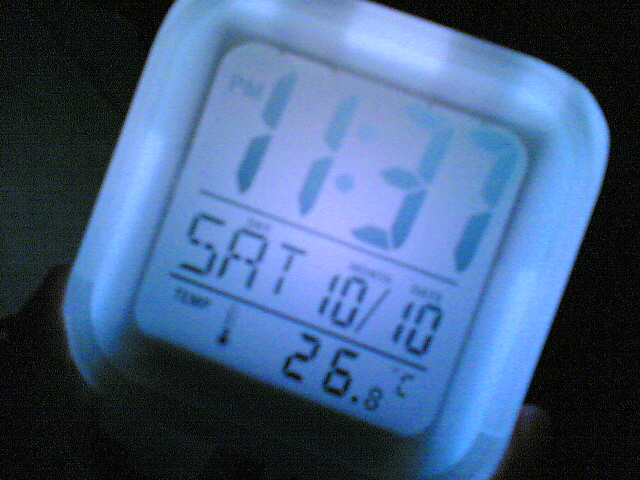In a dark room, possibly a bedroom, this image showcases a close-up of a glowing digital clock with a thick, square-shaped, light blue or white border. The background is entirely black, emphasizing the illuminated clock. The screen displays the time as 11:37 PM in black computerized print, with a line below the time separating it from the date and temperature details. It indicates Saturday, October 10th, with "SAT" and "10/10" respectively. Below the date, the temperature is shown as 26.8 degrees Celsius, alongside an icon of a thermometer partially filled in. The clock emits a glow around its border, casting a slight shadow on the screen, creating a striking contrast against the dark background.